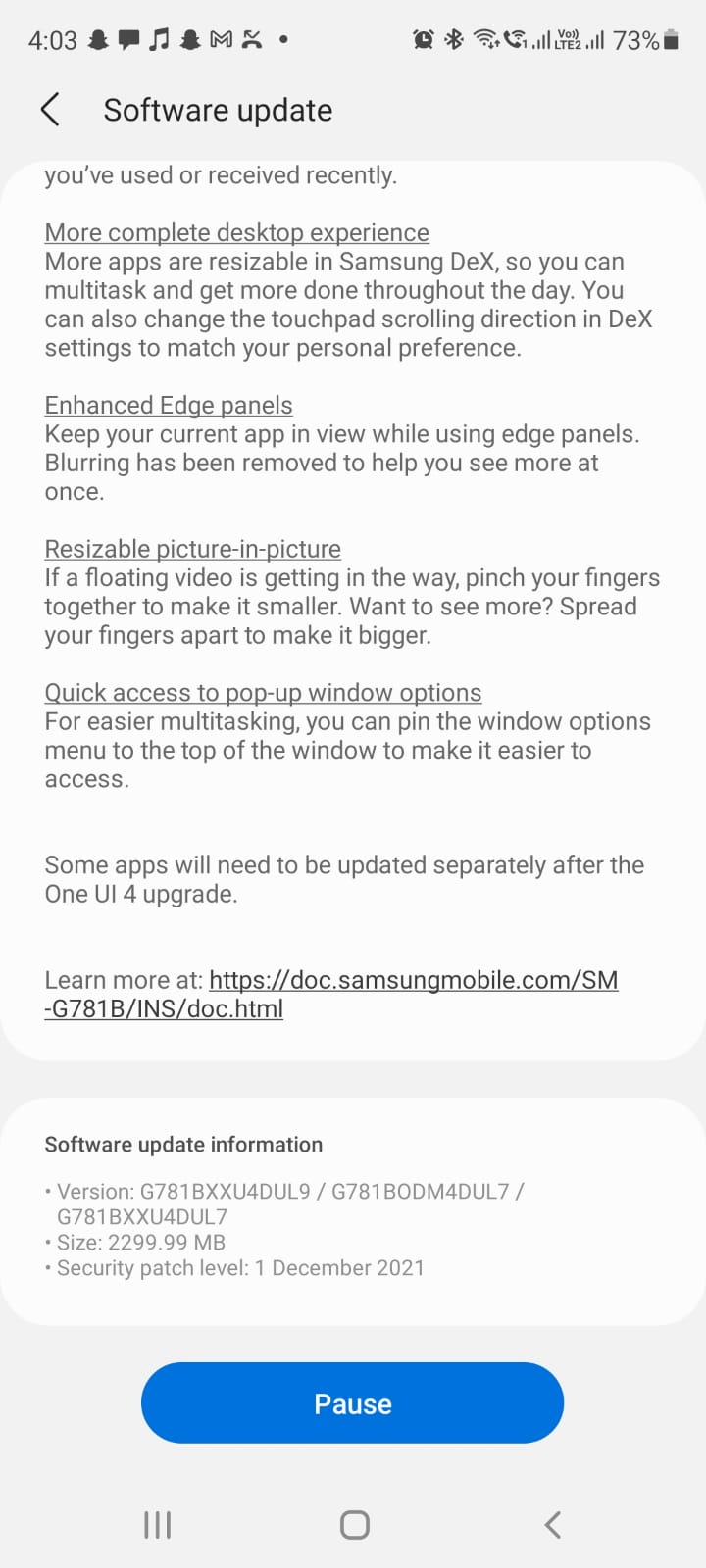This image is a screenshot of someone’s phone displaying a software update notification. At the very top, there’s a gray status bar with black text indicating it’s 4:03 PM and showing a battery level of 73%. Below the status bar, there’s a left-facing arrow accompanied by the text "Software update."

The main section of the image contains a white background with black text, although part of the text is cut off. The visible message reads: "You've used or received recently more complete desktop experience. More apps are resizable in Samsung DEX, so you can multitask and get more done throughout the day. You can also change the touchpad scrolling direction in DEX settings to match your personal preferences. Enhanced edge panels, resizable picture-in-picture, quick access to pop-up window options. Some apps will need to be updated separately after the One UI 4 upgrade. Learn more at," followed by a link to samsungmobile.com.

Beneath this message is a section labeled "Software Update Information," which details the version, size, and security patch level of the update. At the bottom of the screenshot, there’s a large blue button centered on a gray background, with white text that reads "Pause."